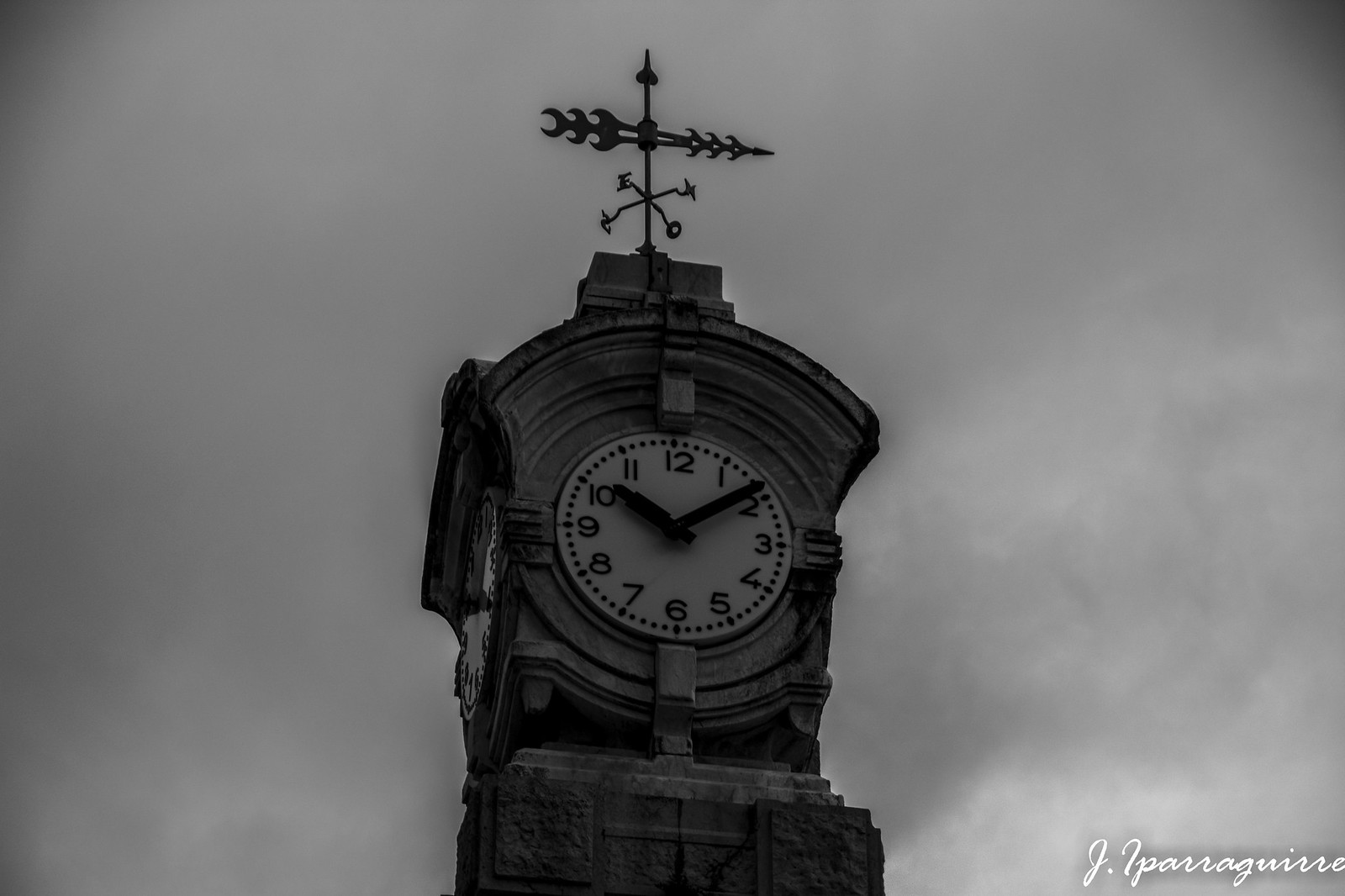The black and white photograph captures a tall clock tower against a cloudy, overcast sky. The clock, which is set at 10:09, features a white face with black numbers from 1 through 12 and minute markings around the edge. Encased in a stone frame, the clock is topped by an elaborate weathervane: an arrow with a crescent moon-shaped tail and directional letters for north, south, east, and west—with west denoted by "O," indicative of the French word "ouest". The building, appearing gray in the monochrome image, also bears a signature in white cursive at the bottom right corner, reading "J. Iparraguirre".